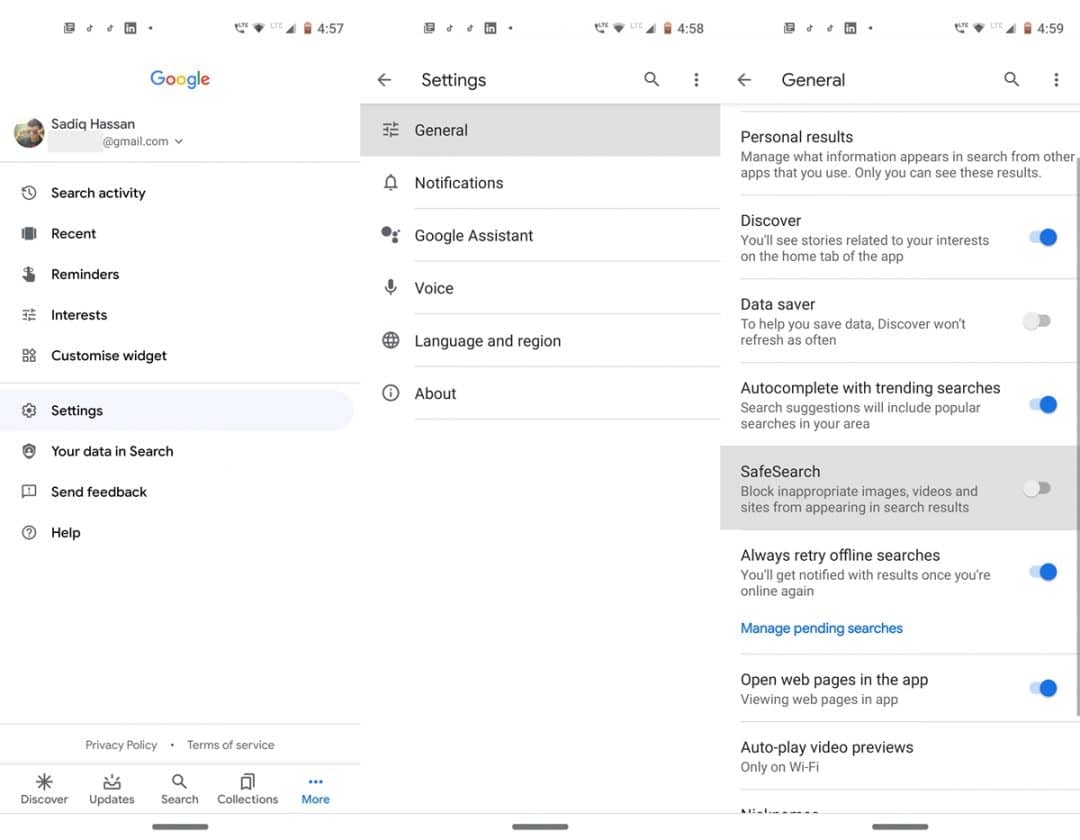This series of screenshots captures various steps of a user named Sadiq Hassan navigating through their Google account settings on a mobile phone. 

In the first screenshot (taken at 4:57 PM), the Google homepage is visible with the iconic Google logo displayed in the top left corner. Sadiq’s profile picture, depicting them standing outdoors wearing a black hat, is shown on the left side of the page along with their name and a partially blurred-out email address ending in "@gmail.com." 

The second screenshot (captured at 4:58 PM) shows that Sadiq has opened the Google account settings page. Various settings options are displayed in the middle of the screen.

In the third screenshot (taken at 4:59 PM), Sadiq navigates to the "General" settings section. The subsequent steps indicate that they are moving towards the "SafeSearch" settings, though it is unclear whether they intend to turn this feature on or off. 

This well-documented sequence, displayed through multiple timestamps, showcases the user systematically managing their Google account settings.